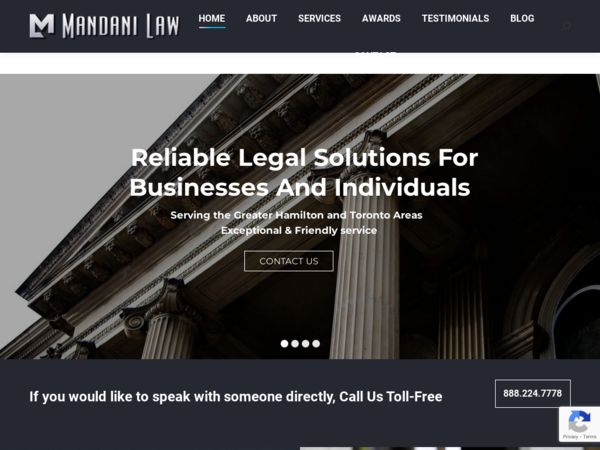This image, sourced from the Mandani Law website, features a prominent black bar at the top, adorned with a sleek silver logo where an 'L' and an 'M' are intricately fused together to represent Mandani Law. Adjacent to the logo, "Mandani Law" is clearly written. Below this header are navigation tabs titled Home, About, Services, Awards, Testimonials, and Blog.

A thin white bar runs beneath the black one, leading to a captivating photograph showcasing the overhang, roof, and ceiling of a distinguished building, such as a courthouse. Majestic grayish-brown columns stand tall in the foreground, emphasizing the structure's grandeur.

The central text within the image declares: "Reliable legal solutions for businesses and individuals. Serving the Greater Hamilton and Toronto areas with exceptional and friendly service," inviting viewers to learn more. A conspicuous "Contact" button is positioned below this message. At the footer, a note encourages direct communication, stating: "If you would like to speak to someone directly, call us toll-free," accompanied by the phone number to the right.